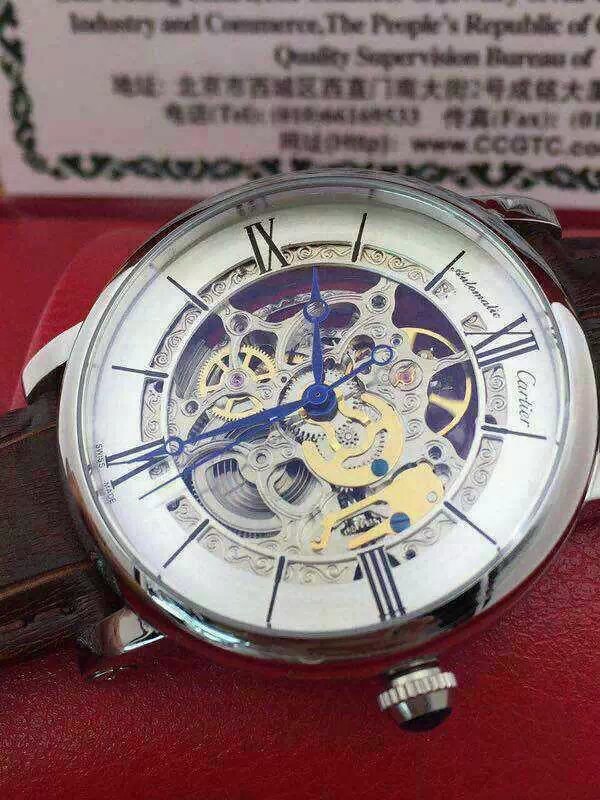This macro photograph showcases a sophisticated Cartier watch with intricate detail. The watch, adorned with a dark chocolate brown leather strap with light brown stitching, is set against a maroon felt background. The silver housing of the watch encloses a white face embellished with silver accents and embroidered edges. Prominently featured are blue Roman numeral hour markers and matching blue hands, currently indicating the time as half past nine. The center of the watch face reveals the intricate mechanism within, displaying golden and silver gears. Behind the watch, a blurry label with both Chinese characters and English text can be discerned, mentioning "Industry and Commerce, the People's Republic of" and "Quality Supervision Bureau of." The finely ribbed silver turn dial adds to the elegance of this meticulously crafted timepiece.